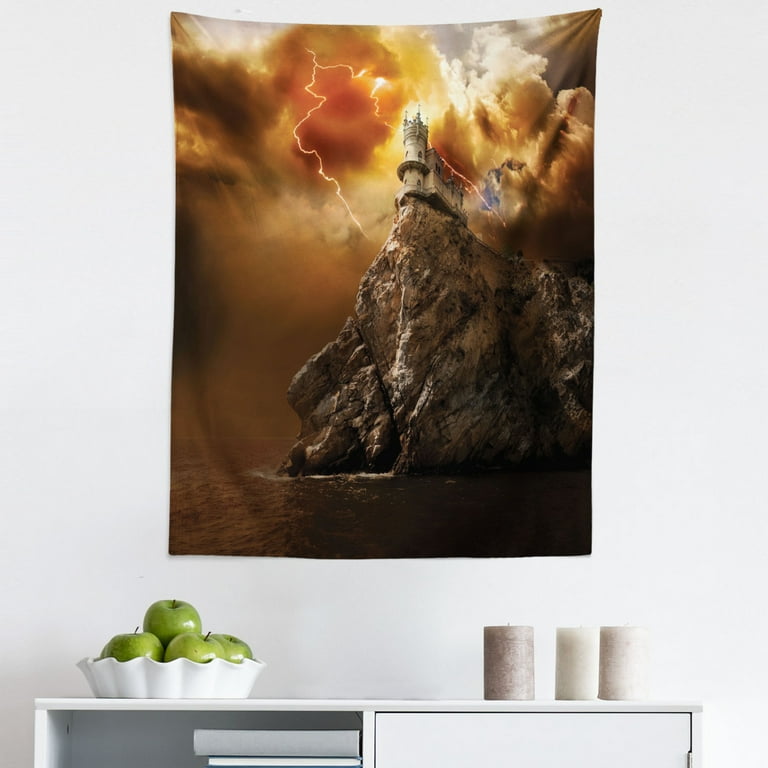The photograph is taken inside a home, showcasing a beautifully arranged scene against a large grey wall. Central to the composition is a striking cloth tapestry depicting a castle perched on the edge of a tall, craggy cliff overlooking a dark, tumultuous ocean. The sky above the castle is stormy, with dramatic lightning bolts slicing through ominous clouds painted in hues of black, orange, white, and dark brown, making for an intense and foreboding atmosphere.

Beneath this vivid tapestry, there is a clean, white table contributing to the serene setup. On the table, a white scalloped porcelain bowl holds green Granny Smith apples, adding a touch of freshness to the scene. Beside the bowl, three chunky pillar candles in shades of white and sandy beige stand neatly arranged. The table also features a book insert section containing two books, further adding to the clean, minimalistic look of the setting.